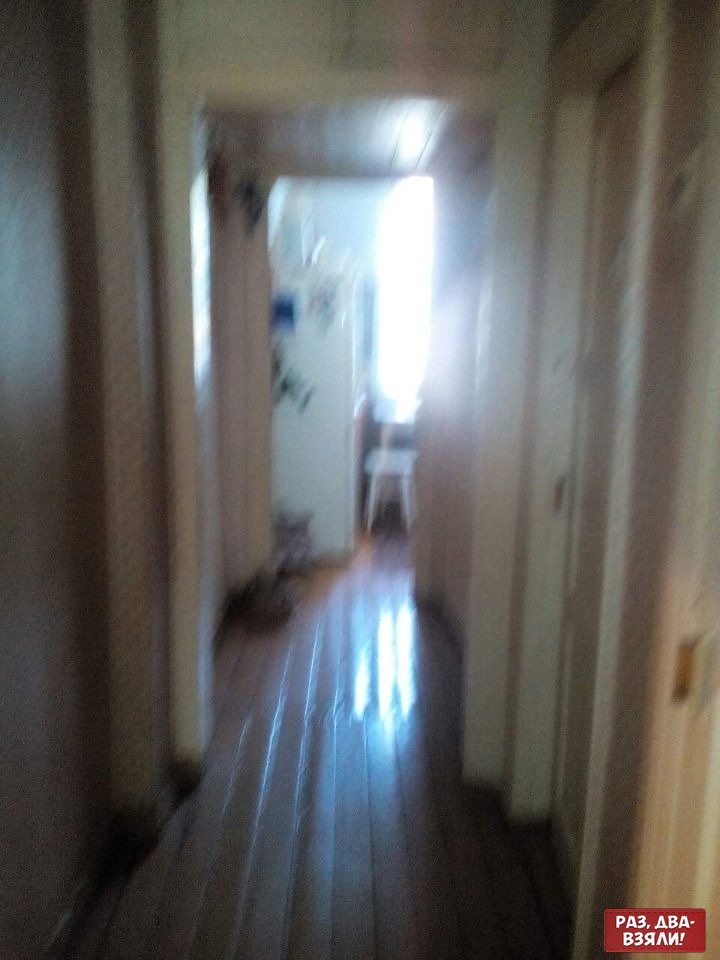This photograph, though blurry and of low quality, appears to have been taken in a residential hallway featuring a wooden plank floor, possibly brown in color, though the distortion makes it difficult to confirm. The flooring seems warped; however, this could also be an effect of the image’s blurriness. The surrounding walls and door frames are painted white. On the right side of the hallway, there are a couple of doorways visible. At the end of the hall, a doorway leads to what seems to be a kitchen. A white, boxy refrigerator is discernible in the distance, with some indistinct items attached to its side.